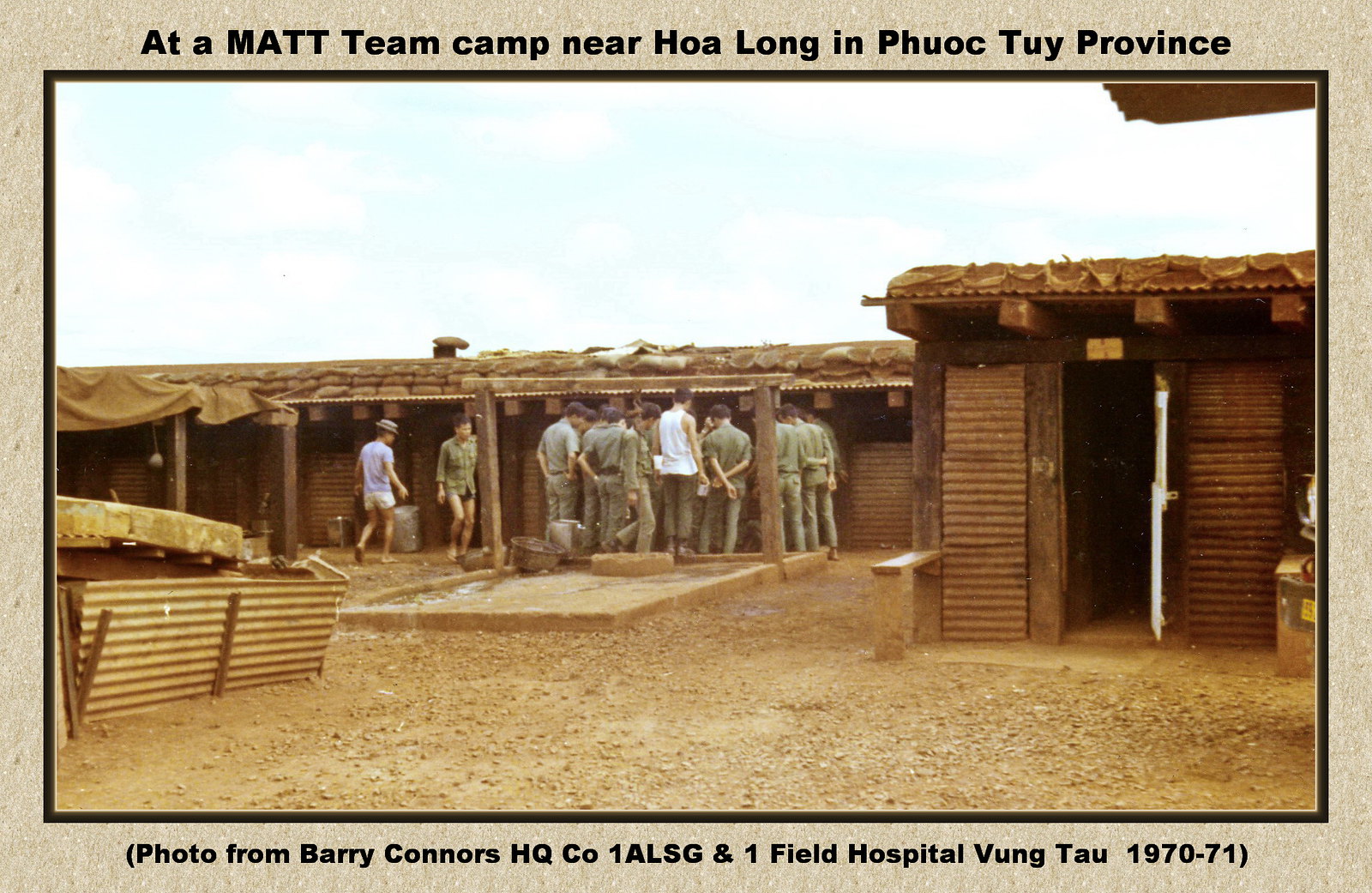This photograph, taken by Barry Connors between 1970 and 1971, captures a military scene at a MATT team camp near Hoa Long in Phuoc Tuy Province. The setting appears to be a military base with a mix of wooden and sheet metal buildings, including a bunker or small structure to the left and a building with an open white door and a bench to the right. In the center background, a decently large group of men in military uniforms, with a few wearing casual clothing like shorts, a white tank top, or a blue T-shirt, huddle together on barren, rocky ground. The sky above them is a muted light blue with some cloud cover, enhancing the austere atmosphere of the scene. The photo's colors are subdued, indicating its age and the gritty nature of the setting. The text above the photograph reads, "At a MATT team camp near Hoa Long in Phuoc Tuy Province," while the bottom text states, "Photo from Barry Connors HQ CO 1 ALSG and 1 Field Hospital Vung Tau 1970-71."